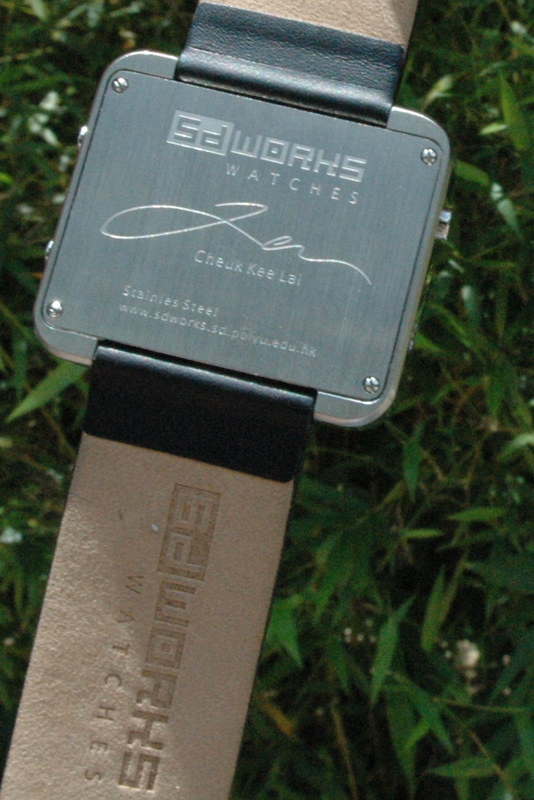This photograph captures the back of a sophisticated smart watch produced by SD Works Watches. The watch, encased in stainless steel, features detailed engravings and labels. Prominently displayed is the maker’s signature, Chuck Kee Lai, with each part of his name clearly distinguished. Additionally, the company's website, www.sdworks.sd.poly.edu.hk, is etched at the bottom. The watch’s side profile reveals a sleek design with visible knobs, and it is complemented by a premium leather strap that also bears the SD Works Watches imprint. The image is taken outdoors in bright daylight, with a green bush subtly blurred in the background, focusing attention entirely on the watch's impeccable craftsmanship.